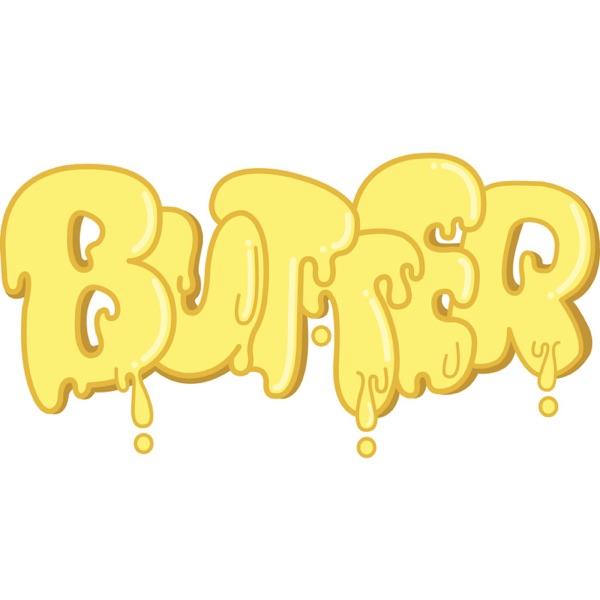The image features the word "BUTTER" prominently set against a white background. Each letter is styled to resemble actual dripping butter, rendered in a vibrant yellow color with darker yellow outlines and shadows for depth. White highlights on the right edges of the letters suggest light reflecting off them. The letters appear thick and cartoon-like, with a playful, slightly chaotic arrangement where they seem to melt and merge together, creating a messy, graffiti-like aesthetic. Below the letters, yellow drips and splotches are visible, enhancing the illusion of melting butter. The scene captures a whimsical, almost surreal depiction of the word "BUTTER" as if it were made from real, melting butter.